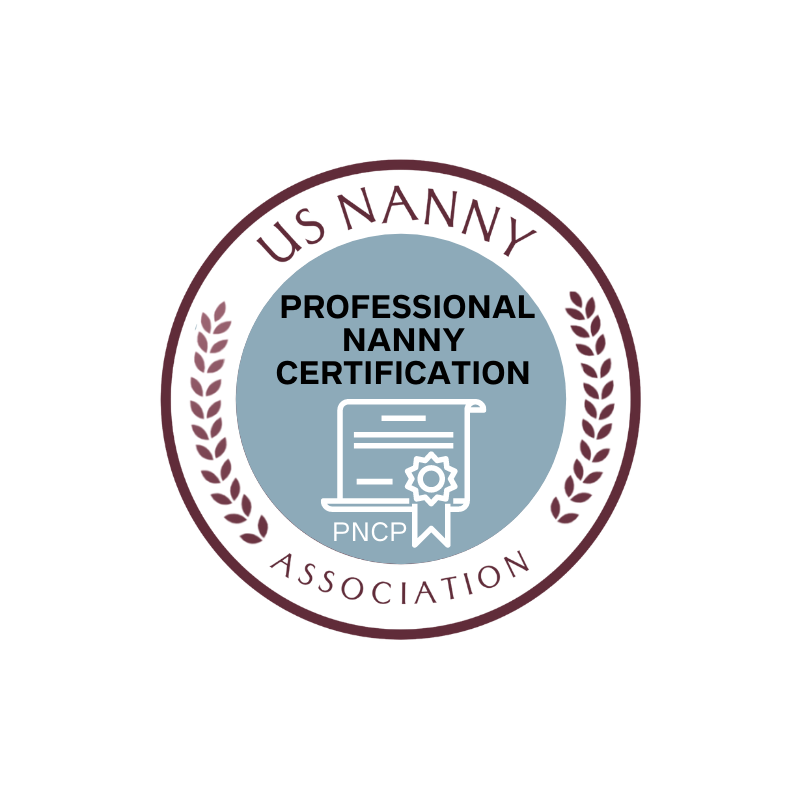The image showcases an intricately designed circular emblem set against a solid white background. The outermost part of the circle features a dark burgundy border. Encircling this border is a white strip with burgundy text, which reads "US Nanny" at the top and "Association" at the bottom. On either side of the text, the white strip is adorned with two clusters of leaves, each group arranged to imply the presence of a twig.

Within the white border lies a medium blue inner circle. At the top of this inner circle, in black lettering, the text reads "Professional Nanny Certification". Below this text, there is an icon depicting a certificate with a ribbon, symbolizing an award or credential. Underneath the certificate icon, the acronym "PNCP" is displayed in capital letters, completing the professional and authoritative look of the emblem.